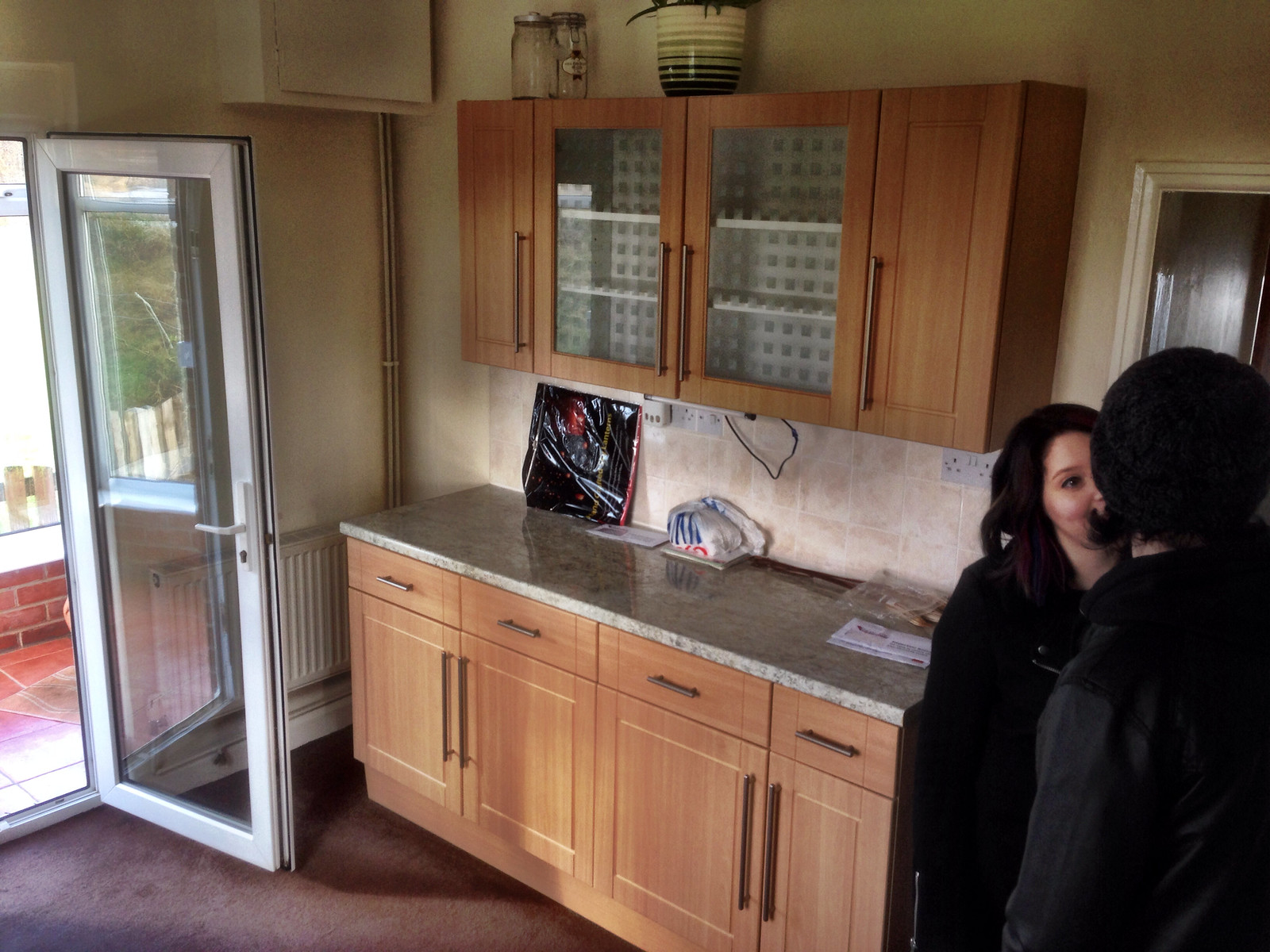In this indoor shot, the scene is set in a modern kitchen with distinctive design elements. To the left, an open glass door suggests a view leading out to possibly a patio area, allowing natural light to seep into the space. The flooring is carpeted, and the right wall features upper cabinets crafted from light brown wood, some with glass-fronted sections that reveal their empty interiors. Below these are sleek white granite countertops extending over four matching lower cabinets.

Two young individuals are the focus of the image, positioned towards the lower right. Both are dressed in dark attire, reminiscent of a gothic style, evoking a mysterious and somewhat brooding atmosphere. The young man, identifiable by his long hair peeking out from under a skullcap, has his back to the camera, obscuring his face. Opposite him, the young woman, partially visible with her right eye and side of her face in view, appears engaged in conversation, her head slightly tilted. The subdued tones and fashion choices suggest an intense or deep dialogue shared between them.